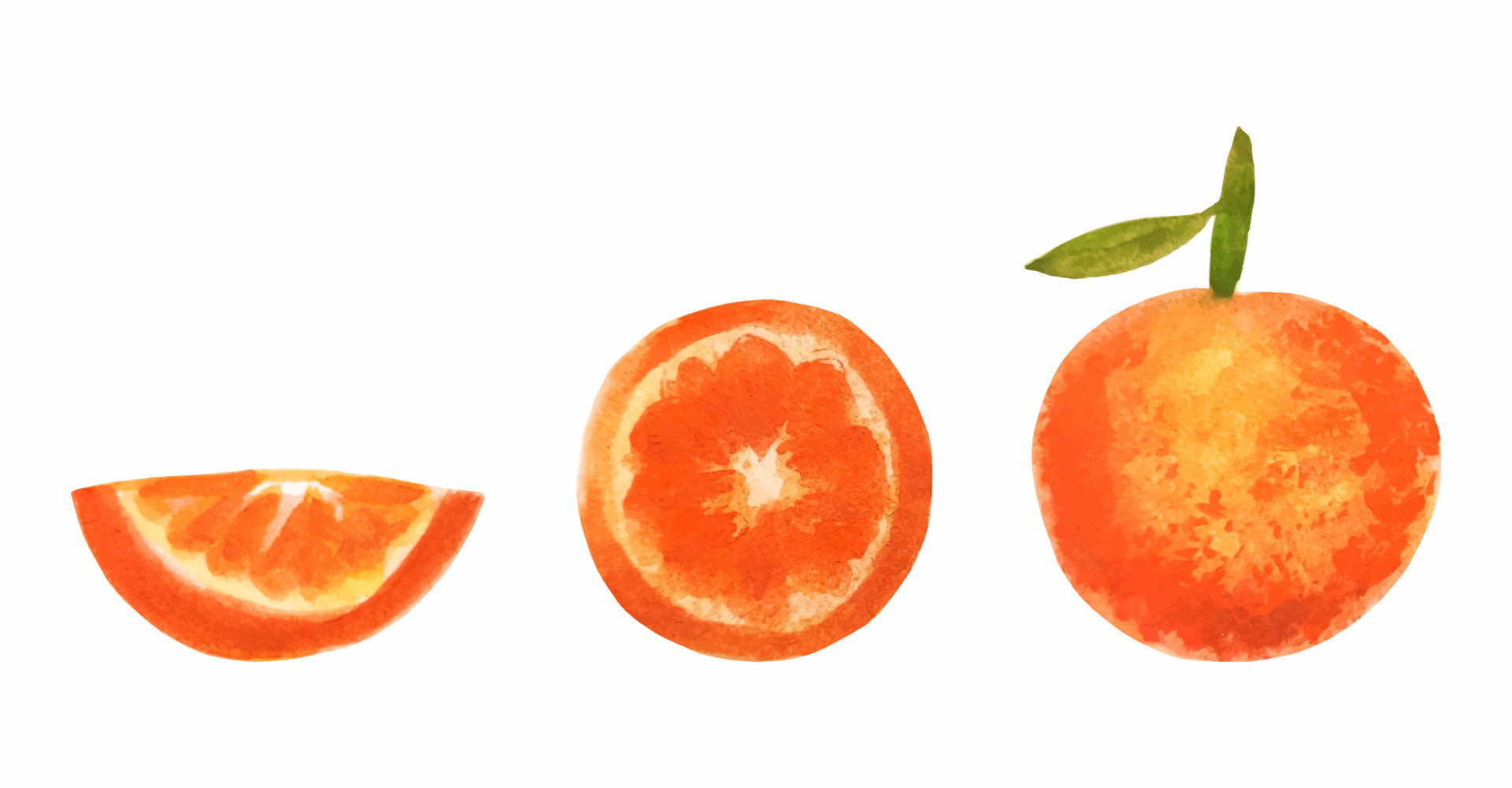This illustration consists of three distinct images of an orange, each rendered in a style reminiscent of charcoal with watercolor-like effects. The background is pure white, accentuating the vivid yet softly blended colors of the fruit. 

On the far left, there is a single orange slice with its rind forming a partial arc, exposing the vibrant orange flesh above it. The middle image features an orange cut in half, displaying the inner structure with segments radiating outwards from a central white core. 

Finally, on the far right, a whole orange is depicted, complete with a small green stem and two leaves—one pointing upward and the other extending to the left. The rind of the whole orange showcases a rich array of colors, ranging from pale yellow to deep red-orange, giving it a textural, mottled appearance. The overall style is simplistic with a loose, fuzzy quality around the edges, contributing to its watercolor-like charm.